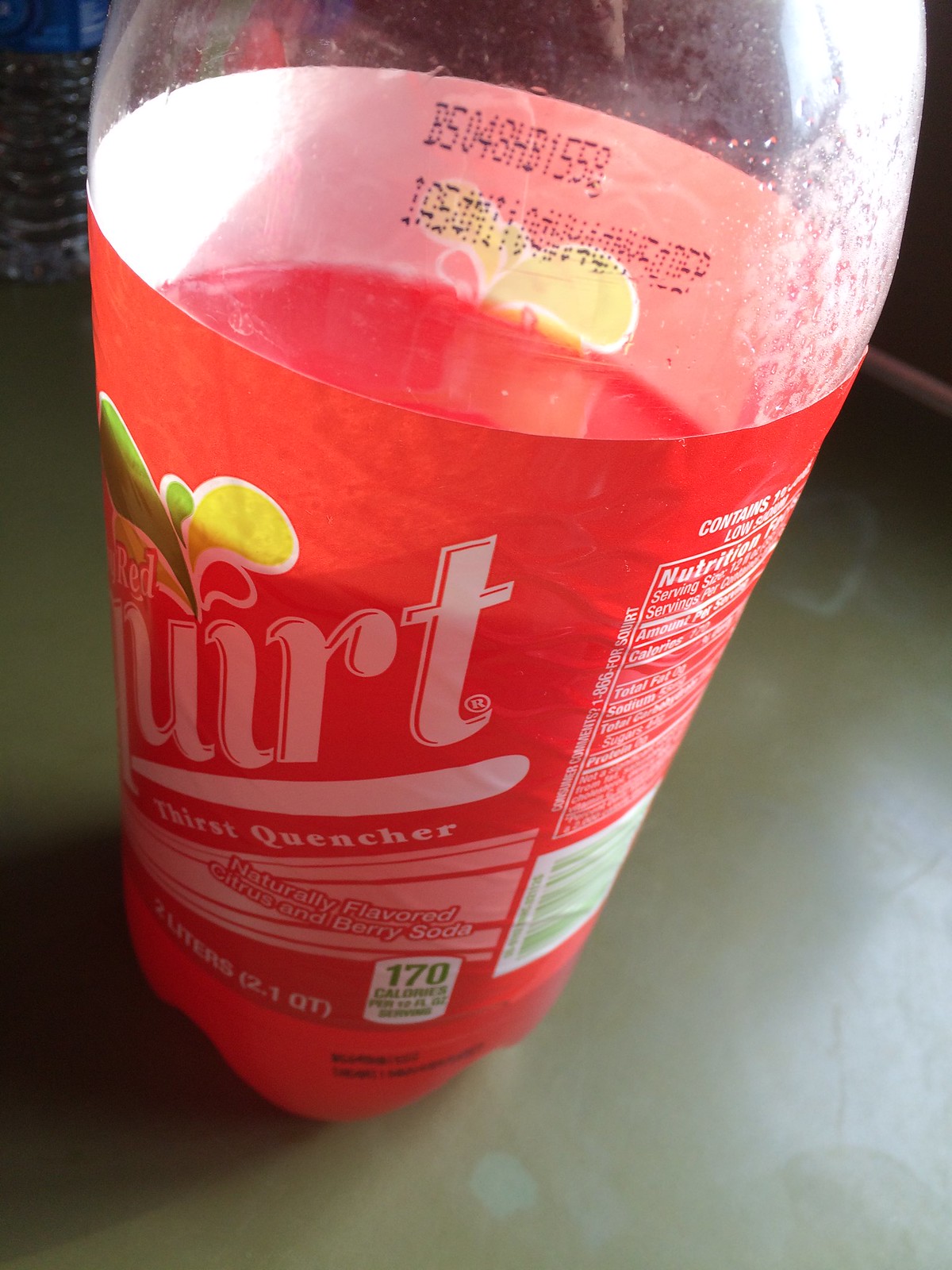This color photo showcases a close-up of a two-liter clear plastic bottle of Red Squirt soda, which is filled approximately two-thirds with a pinkish-red liquid. The bottle features a prominent orange-red label that reads "Red Squirt Thirst Quencher" with an additional description: "naturally flavored citrus and berry soda." The label's text is predominantly white and also includes vibrant colors of yellow, orange, and green, particularly around the brand name. A small, square white field near the center of the label mentions "170 calories," though the fine print is blurred and unreadable. The image, taken from an angle, reveals parts of the nutritional information on the back of the bottle and a barcode at the lower section of the label. The bottle is placed on a greenish-gray flat surface, with the sunlight reflecting off the liquid and creating a glare on the label. The entire setup gives the impression of the bottle and the surface inclining slightly downhill towards the right side of the frame.